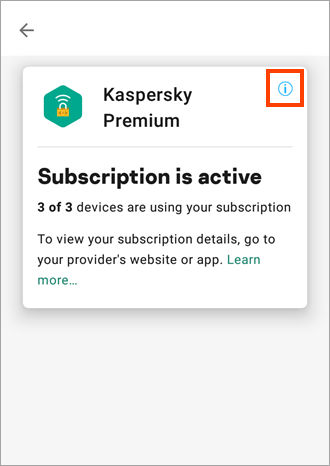Here is a detailed and cleaned-up caption for the described image:

---

A screenshot of the Kaspersky Premium application is displayed, highlighting an active subscription notification. This subscription is currently utilized by three out of three authorized devices. For further subscription details, users are prompted to visit the provider's website or app via the "Learn more" hyperlink, which is distinctly marked in blue. 

To the left of the notification, the Kaspersky logo is prominently featured. The logo consists of a blue hexagonal shape enclosing a lock symbol, with what appear to be Wi-Fi signals emanating from the lock. The entire notification is set against a clean white background, and the text is primarily in black, apart from the blue hyperlinks which offer additional information upon being clicked. 

In the upper right corner, there is a blue information icon ("i") that users can click for basic information and further support from Kaspersky's website.

---